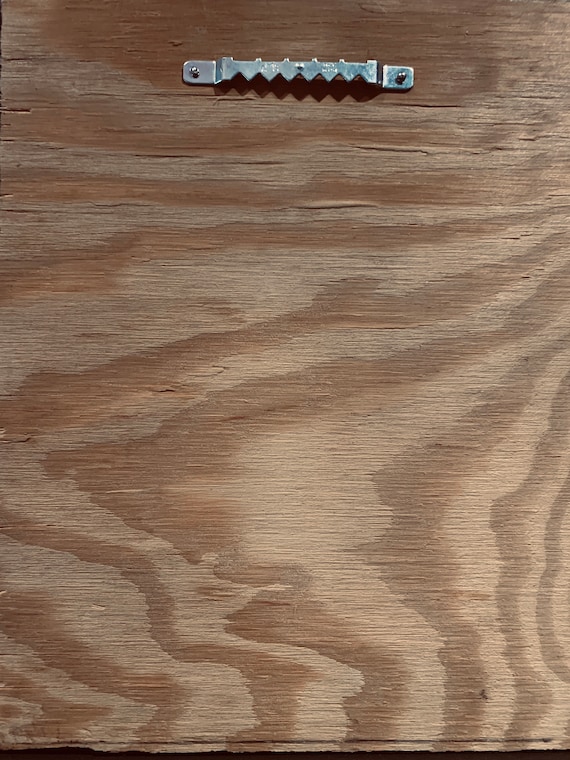The image depicts the back of a wooden frame or board, characterized by a flat, solid plywood surface that exhibits light tan to light brown shades, accented with subtle, wavy horizontal grain patterns and marbling in darker, reddish-brown hues. Positioned at the top of the frame, a serrated, silver metal hanger is attached to the wood, secured by two small screws, one on each side. The jagged, toothed part of the hanger protrudes slightly outward in a manner resembling a saw blade or a "C" shape, indicating its purpose for wall mounting. Additionally, there is a noticeable black line at the bottom of the image, potentially drawn with a pencil for measurement or cutting purposes.